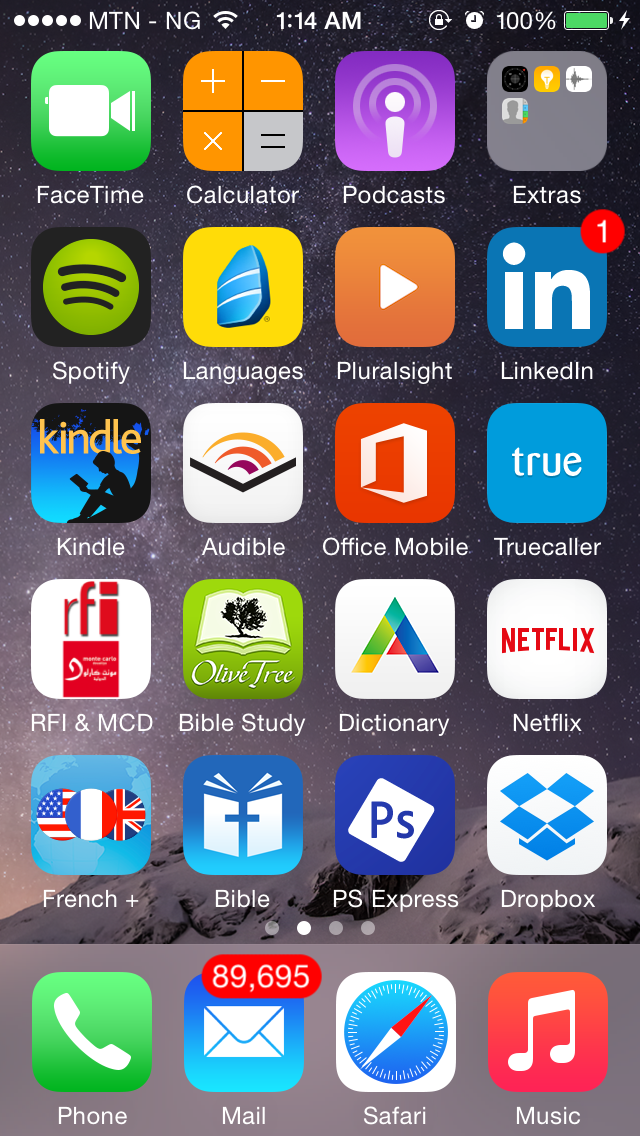This image displays a screenshot of a tablet's home screen, neatly arranged into four columns and six rows, showcasing a total of 24 app icons. In the first row from left to right, the apps are FaceTime, Calculator, Podcasts, and Extras. The second row features Spotify, Languages, Pluralsight, and LinkedIn. The third row hosts Kindle, Audible, Office Mobile, and Truecaller. In the fourth row, you will find RFI and MCD, Olive Tree Bible Study, Dictionary, and Netflix. The fifth row includes apps labeled French, depicted with American, French, and British flags; Bible, represented by an open book with a cross; PS Express; and Dropbox, with its recognizable blue box icon. The sixth row houses the essential apps for Phone, a green button with a white telephone icon; Mail, represented by a blue background with a white envelope and an overwhelming 89,695 unread emails; Safari, symbolized by a compass icon; and Music, characterized by a red background with an eighth note sign.